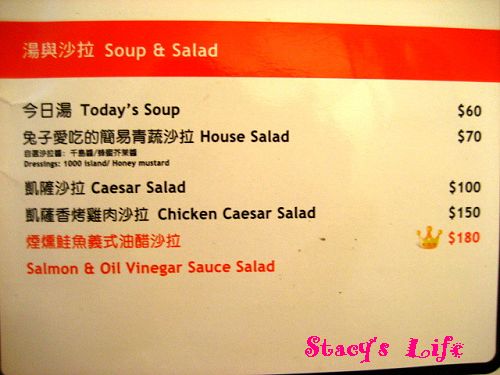The image is a vibrant, color photograph featuring an illuminated sign inside a restaurant. The sign itself is predominantly white, with a distinctive orange or red band across the top that includes four Chinese characters along with the English wording "Soup & Salad." This strip establishes the section's theme.

Below this band, the sign is neatly organized with black text. At the top, there are three Chinese characters followed by the English phrase "Today's Soup," priced at $60, potentially in Hong Kong dollars. Underneath, more Chinese characters appear next to "House Salad," priced at $70.

Continuing down the sign, there is a mention of different salad dressing options, listed as "1,000 Island / Honey Mustard." Underneath that, four Chinese characters introduce "Caesar Salad," which costs $100. Below this line, more Chinese text labels "Chicken Caesar Salad," priced at $150.

At the bottom of the sign, a section in orange text includes Chinese characters next to a yellow or golden crown symbol, followed by a price of $180. The final item listed is "Salmon & Oil Vinegar Sauce Salad."

The image is watermarked in the bottom-right corner with the phrase "Stacy's Life in Pink," suggesting that this photo was posted on Stacy's blog.